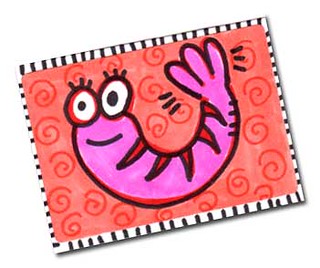The image appears to be a cartoon poster or sticker with a black and white striped border surrounding a red background adorned with darker red swirls that form intricate patterns, almost resembling the letter "E." The central figure is a whimsical, pink, watercolor or colored-pencil drawn character that resembles a cross between a seal, shrimp, and earthworm. The character has a U-shaped body and is decorated with five red stripes along its back. It features large white eyes with black pupils and three distinct eyelash lines above each eye. Its tail splits into three sections with streaks that give an impression of movement. A simple, black-line smile graces its face, adding to its charming, albeit somewhat curious appearance.